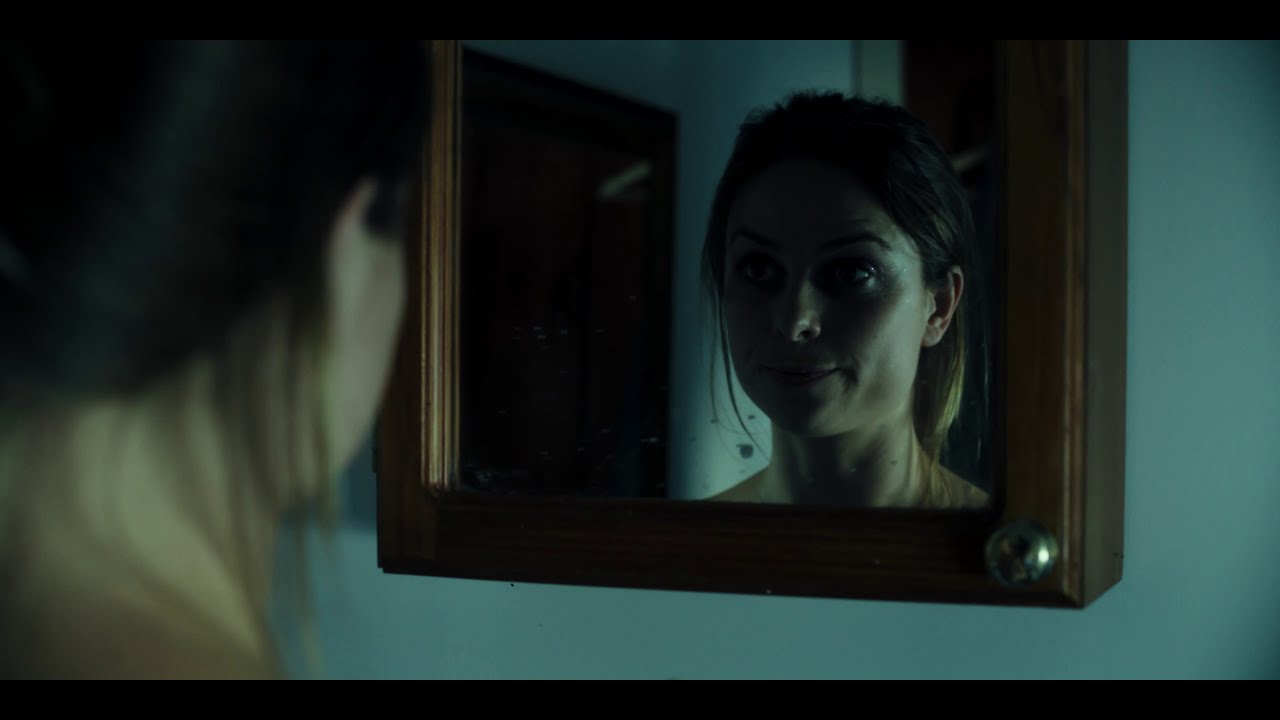This is a wide rectangular photograph of a young woman in her 20s looking at herself in a square mirror that is set in a dark brown wooden cabinet. The photograph has thin black rectangular borders at the top and bottom. The woman, who has light skin, is situated on the left side of the image with the back of her head and hair visible. Her dark brown hair, adorned with blonde highlights and wisps falling near her neck and shoulders, is partly pulled up in a bun. The mirror, slightly to the right of the center, reflects her face with a surprised expression and a closed mouth. Her face is partially covered by a dark shadow. The cabinet on which the mirror is mounted has a silver knob in the bottom corner and is affixed to a light turquoise wall. Additionally, the reflection in the mirror shows part of the cabinet’s dark brown border and to the left side of the mirror, a brown doorframe. Only the woman's head and the back of her neck are visible, as the rest of her body is cropped out of the shot.